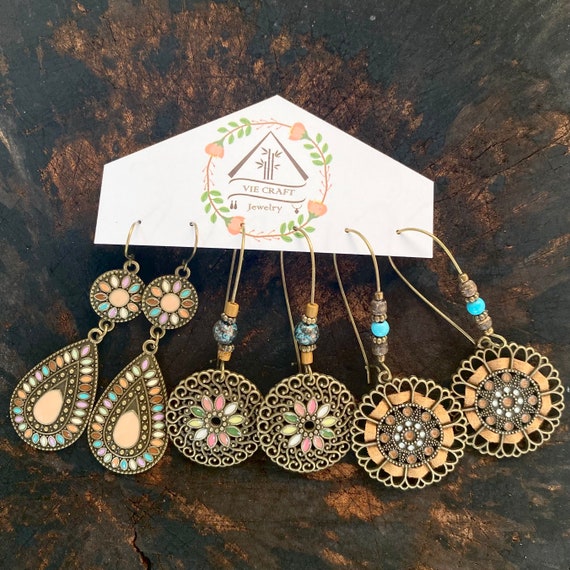This image is an advertisement for a set of beautifully handmade earrings by ViCraft Jewelry. The photograph shows three pairs of unique, dangle earrings displayed on a cardboard piece shaped like a pentagon or trapezoid. The card features a logo with orange flowers and green leaves, adorned with the brand name, ViCraft Jewelry. The entire display rests on a warm, camel-brown wooden surface with a black, marble-like pattern.

From left to right, the first pair of earrings features a combination of a circular dangle with a teardrop shape beneath it, embellished with vibrant multicolored gems—turquoise, lavender, cream, orange, and brown. The middle pair showcases an ornate floral design framed by circular filigree, incorporating pink, coral, dark green, lime green, and white gemstones. The third pair is circular, decorated with orange, cream, and black elements, and accented with turquoise beads near the hooks. Each pair of earrings has a metal base, predominantly a duller gold or copper color, and presents a tribal-inspired aesthetic with intricate floral designs and various colorful jewels. The diverse shapes and colors make this set a visually striking and versatile collection.